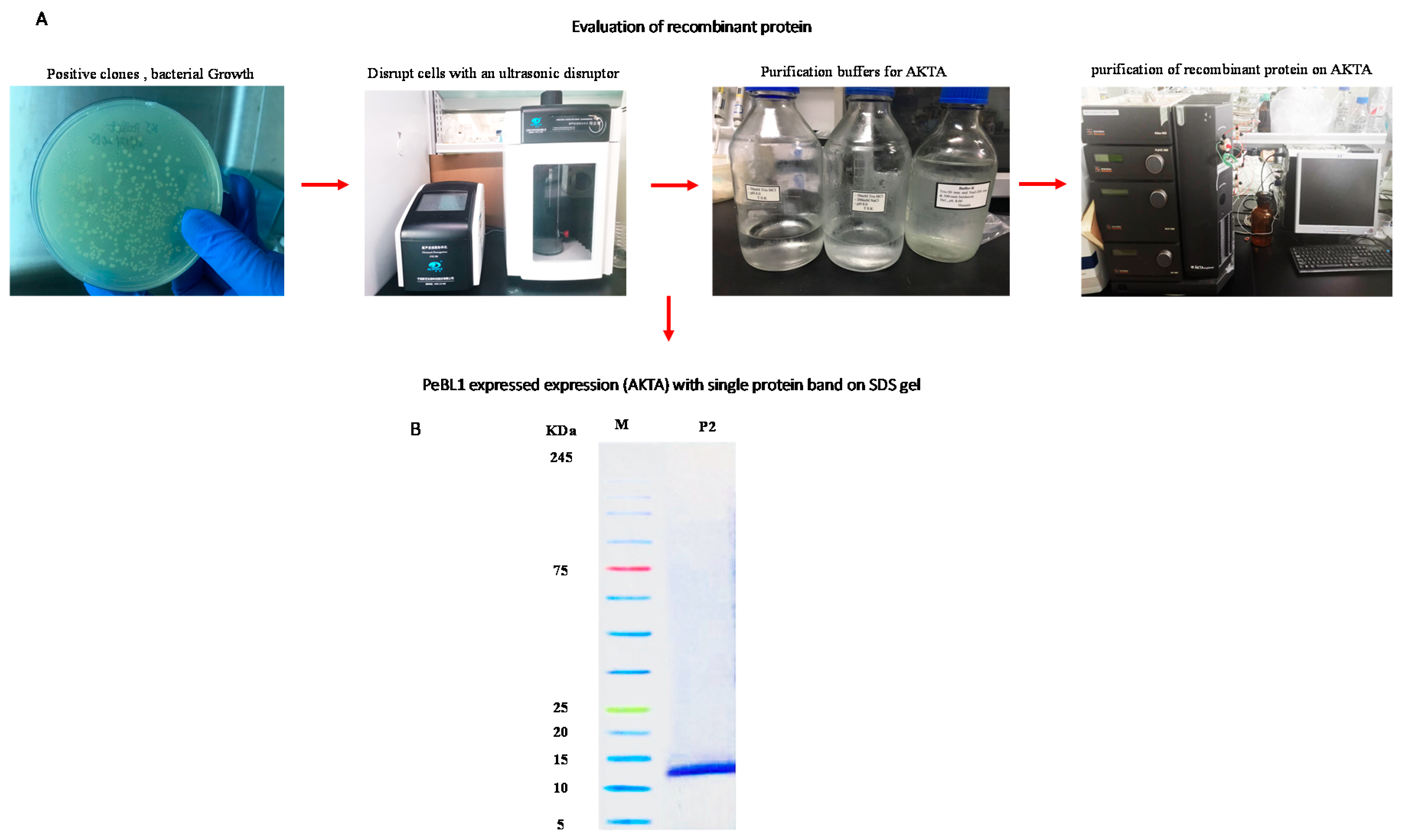The diagram, titled "Evaluation of Recombinant Protein," details a step-by-step procedure for protein analysis through a series of scientific photographs labeled from A to B. The process starts at the top-left with image A, which shows a round petri dish containing positive clones of bacterial growth being handled by a scientist wearing latex gloves. A red arrow points to the right, continuing the sequence to an image depicting the disruption of cells using an ultrasonic disruptor. This is followed by another red arrow leading to three clear bottles with blue tops labeled “Purification Buffers for AKTA.” The final image on the right shows the “Purification of Recombinant Proteins on AKTA,” involving advanced scientific equipment believed to log data and measure protein expression. A red arrow then directs downwards to a section labeled B, which focuses on "PEBL1 Expression with a Single Protein Band on SDS Gel," indicating the successful expression and visualization of the recombinant protein. Each step is meticulously captured and visually connected with arrows to guide through the evaluation process.